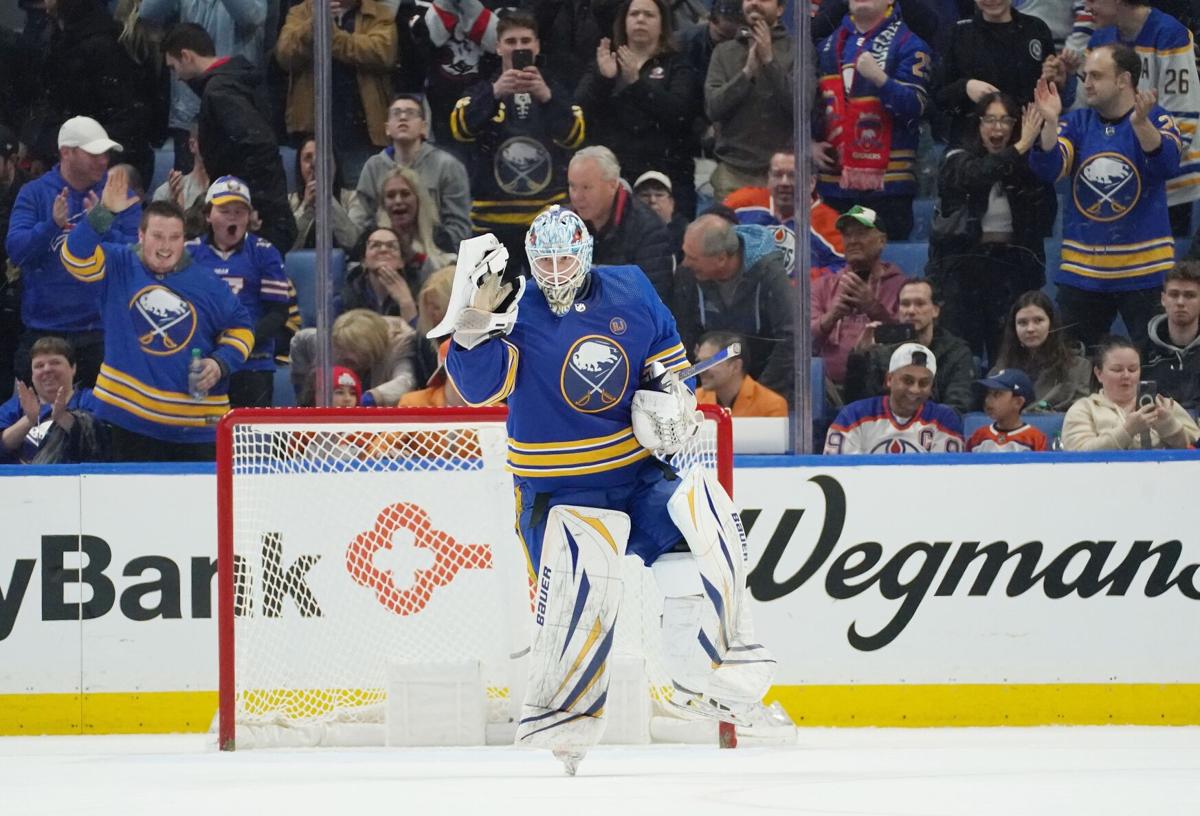This detailed horizontal rectangular photo captures an ice hockey game featuring a fully-equipped goalkeeper in a blue and yellow uniform with white padding, standing by a red frame that holds a white net. He's wearing a white helmet and protective gloves. Behind him, there's a white wall with a yellow stripe at the bottom and a blue stripe at the top, adorned with partially visible advertisements displaying the words "Bank" and "Wegmans." Spectators, dressed mostly in blue jerseys with white buffaloes and yellow stripes, are seen through panels of plexiglass or thick plastic. The fans are actively engaged, with some clapping, taking photos, and others simply enjoying the game. The overall atmosphere is vibrant and lively.